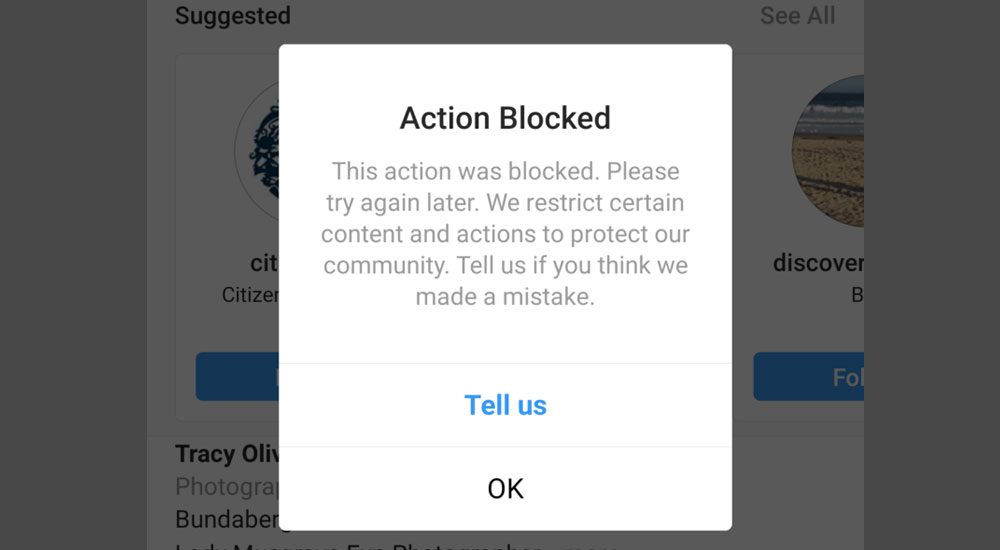The image depicts a web browser page with a prominent "Action Blocked" notification occupying most of the screen. In the background, partially obscured by the pop-up, is a website section that appears to be dedicated to photography, possibly labeled as "Photography" with some additional text that is not fully visible due to the overlay. The notification itself is a large white box with bold black text stating "Action Blocked" and an explanatory note in smaller, gray font that reads, "This action was blocked. Please try again. We restrict certain content and actions to protect our community. Tell us if you think we made a mistake." Below this message are two clickable options: one to report the potential mistake and another labeled "OK" to dismiss the notification and return to the previous page. This suggests that the user was attempting to interact with or contribute to the page, such as by making a comment or adding content, but their action was halted by the platform's content moderation systems.